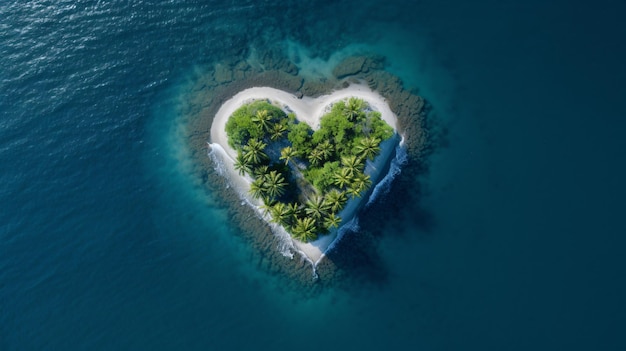This is a highly detailed, photorealistic, AI-generated overhead view of a heart-shaped island set in the middle of a vast blue ocean. The island's perimeter is lined with a ring of rocks visible through the clear tropical waters. Just inside the rocky boundary lies a pristine heart-shaped beach of white sand. Further inward, a dense copse of approximately 25 to 30 green palm and tropical trees forms yet another heart shape. Light reflections in the upper left corner suggest sunlight streaming in from that direction, illuminating the scene. Gentle waves lap against the island's shores, particularly noticeable on the left and right bottom edges. The lack of any visible fish, creatures, or other signs of life enhances the island’s secluded and serene appearance.